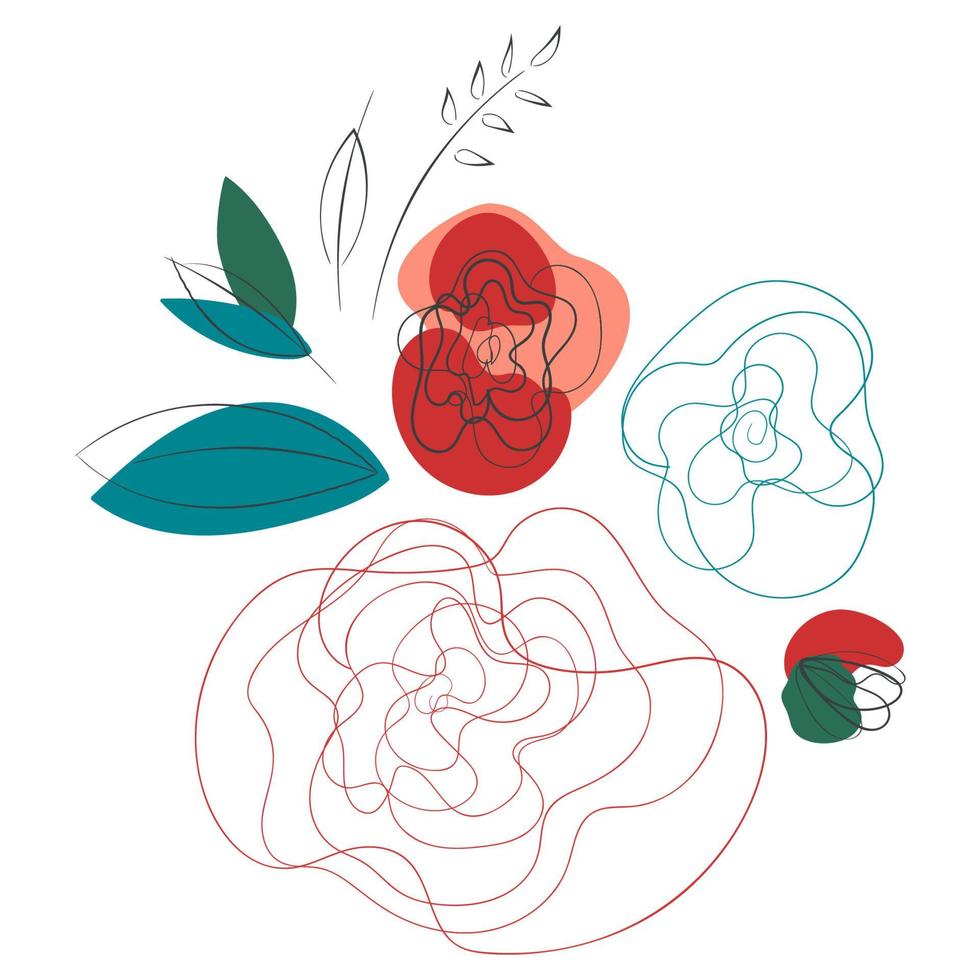The artwork is a simple yet abstract floral piece set against a plain white background, featuring a multitude of diverse elements. In the upper left corner, there is a black-bordered leaf whose fill extends outside the lines. Beside it, a teal leaf sits adjacent to a dark green leaf that points upward. To the right of these leaves lies the outline of another leaf, and further right, a curved line resembling a stem with teardrop-shaped leaves radiating from it. Below this stem, there are overlapping black squiggle marks and two red dots, the larger of which has a pink background. The various elements come together to form an intricate and colorful composition of abstract flowers and leaves, rendered in shades of teal, green, red, black, and pink, with additional blue scribble spiral shapes adding a whimsical touch to the piece.